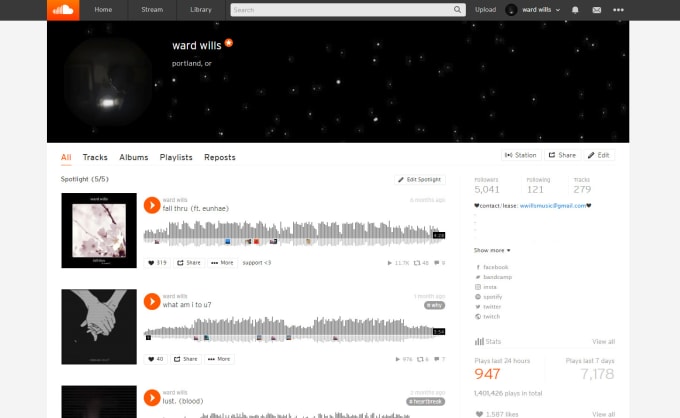This is a screenshot of a desktop or laptop computer screen displaying the SoundCloud profile of an artist named Ward Willis from Portland, Oregon. At the top of the page, there is a dark gray banner featuring the SoundCloud logo in orange and white, along with navigation buttons labeled Home, Stream, Library, Search, Upload, and Ward Willis, indicating that the user is likely logged into Ward Willis's own account.

Just below the banner, there is a black-and-white cover photo with star patterns, showcasing the artist's name and a brief description. Underneath this header, a series of buttons allow navigation through different sections such as All Tracks, Albums, Playlists, and Reposts.

The main section of the page lists several tracks, each with a play button beside it. Key tracks highlighted include "Fall Through" featuring Linne, "What Am I to You?", and "Lost Blood." The artist's statistics are also displayed: Ward Willis has 5,041 followers, is following 121 users, and has 279 tracks available. The profile also shows detailed play metrics, with 947 plays in the last 24 hours and 7,178 plays over the past seven days.